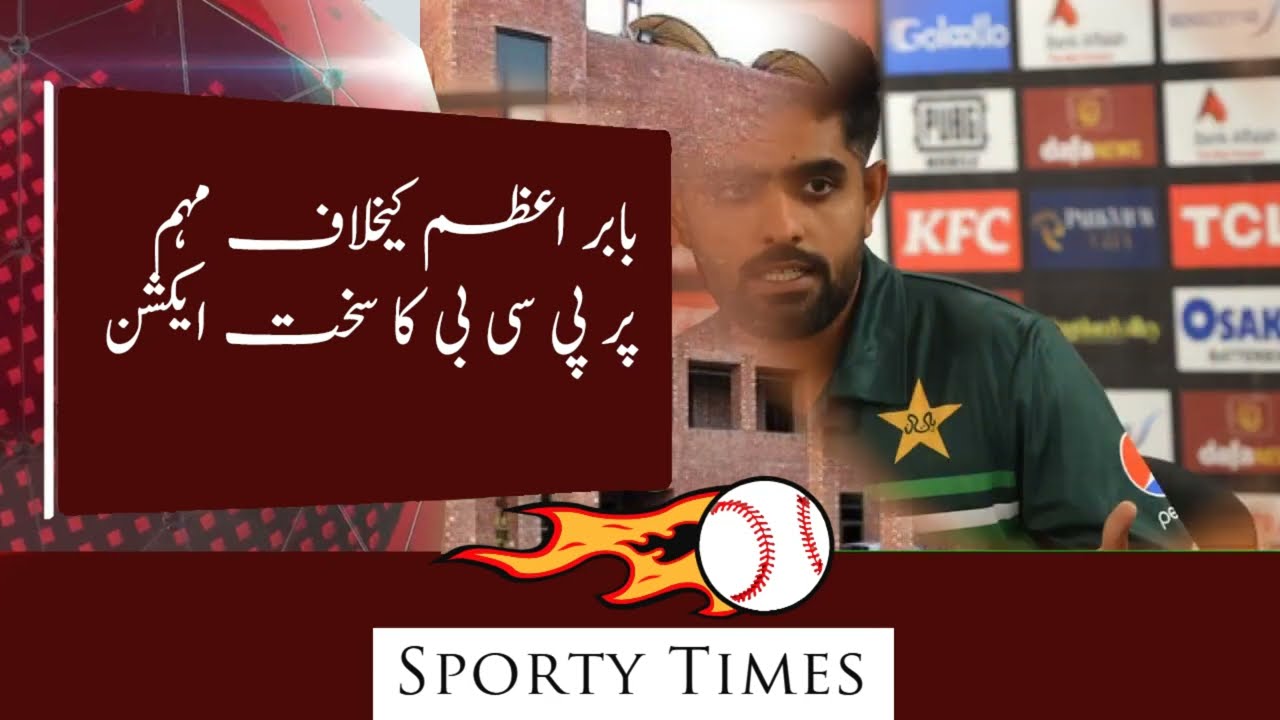The rectangular poster features a predominant maroon palette and displays a collage centered around a focused man with a light beard and mustache, dressed in a green shirt adorned with a yellow star and the Pepsi logo on the left sleeve. Portions of the man are intact while others fade into elements of the background, creating a blended photo-collage effect. His right side merges into an image of a brown building with windows and entryways.

Adjacent to the man, a grid of vibrant, multicolored advertisement signs is visible, displaying various place names such as KFC in white and OSAK in blue. The colors range from pink and white to red, blue, gold, and orange. There are approximately 13 signs on the wall, adding to the visual clutter.

Dominating the right side of the poster is a large dark maroon rectangle with foreign text, possibly in Urdu. Central to the poster is a dynamic illustration of a white baseball with red stitching, trailing flames as if moving at high speed, positioned above a banner with the text "SPORTY TIMES" in black capital letters. The entire composition conveys a vibrant and fast-paced atmosphere, possibly related to sports or baseball.